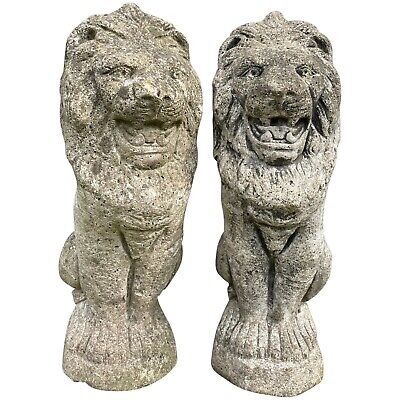This image showcases two weathered stone lion statuettes, likely carved in the late 1800s or early 1900s. The lions are perched upright on small round pedestals, positioned side by side, just inches apart. Both lions, though slightly different in color with the left one showing a hint of beige and the right one being grayer, are nearly identical in design. They are depicted with their front legs straight and their heads held high, facing forward. Each lion features an intricately carved mane, large noses, and slightly open mouths showing worn-down fangs. Their eyes are wide open, giving them a lifelike appearance. The stone used appears to be granite or a similar material, contributing to their aged, pockmarked texture. Despite their stoic posture, there is a subtle, almost anthropomorphic quality to their expressions, as if they are smiling. The background is stark white, enhancing the timeless, almost ethereal quality of the statues, which might have once adorned the steps or entrance of an old building.